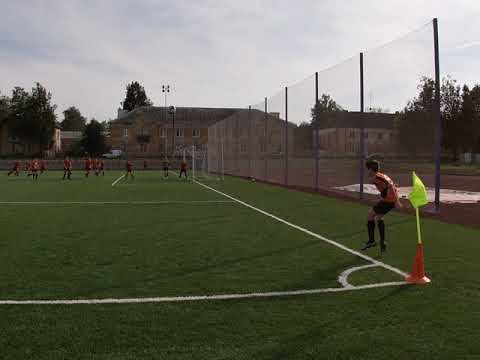The image is a nearly square photograph capturing a vibrant outdoor soccer scene. Predominantly featuring a lush green field marked with crisp white lines, the photo is taken from the corner of the field. Closest to the camera, a young player is poised in an orange shirt, black shorts, and long black socks, standing next to an orange cone topped with a yellow flag, suggesting he is preparing for a corner kick. In the background, a dozen or more children, also dressed in orange uniforms, are actively engaged in the game, with a small soccer net visible in the distance. The field is bordered by a very high chain-link fence, approximately 20 feet tall. Beyond the fence, there are two large buildings, likely schools or office buildings, with one appearing to be multi-story and brick with a gray roof. The backdrop is completed by a mix of green trees, a blue sky with light cloud coverage, and the overall lighting suggesting a slightly overcast yet sunny day.